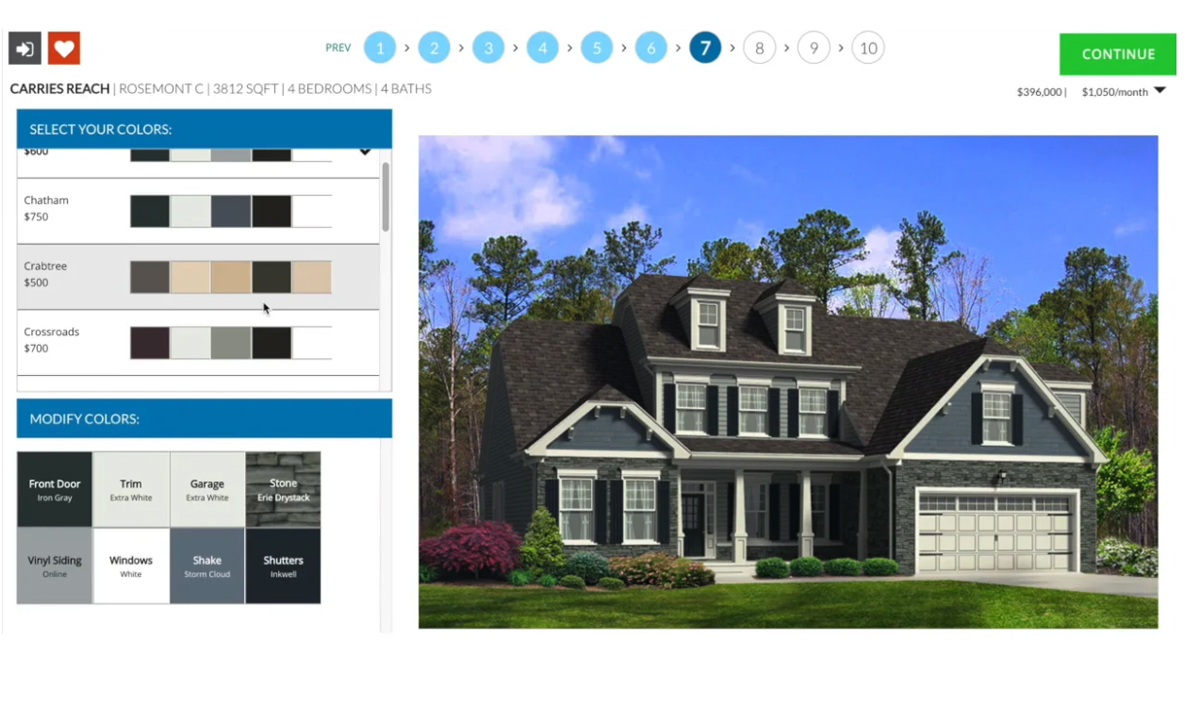A detailed screenshot image caption could be:

"The screenshot displays a sophisticated hybrid interface combining real estate and home customization services. Dominating the top-left corner, the header reads 'Carrie's Research, Rosemont,' highlighting a property with 3,812 square feet, comprising four bedrooms and two bathrooms, firmly establishing the real estate context. The property is listed for $396,000 or $1,050 per month. To navigate, there are numbered bubbles indicating page listings, with the current view being page seven.

On the right side, a high-quality image showcases a beautiful two-story home featuring a high gable roof, a two-car garage, and a charming gray stone facade with a welcoming porch.

Adding an intriguing twist, the left panel is dedicated to home customization options, possibly hinting at home painting services. It presents several color options: 'Chatham - $750,' 'Crabtree - $550,' and 'Crossroads - $700,' accompanied by color swatches. Additionally, there is a customizable menu below allowing changes to the 'front door, vinyl siding, trim, windows, garage, shakes, stone, and shutters,' suggesting an interactive feature akin to a real estate simulation or virtual design tool.

Overall, the blend of real estate listing with home customization elements creates an immersive and potentially innovative user experience, blurring the lines between home buying and virtual design."